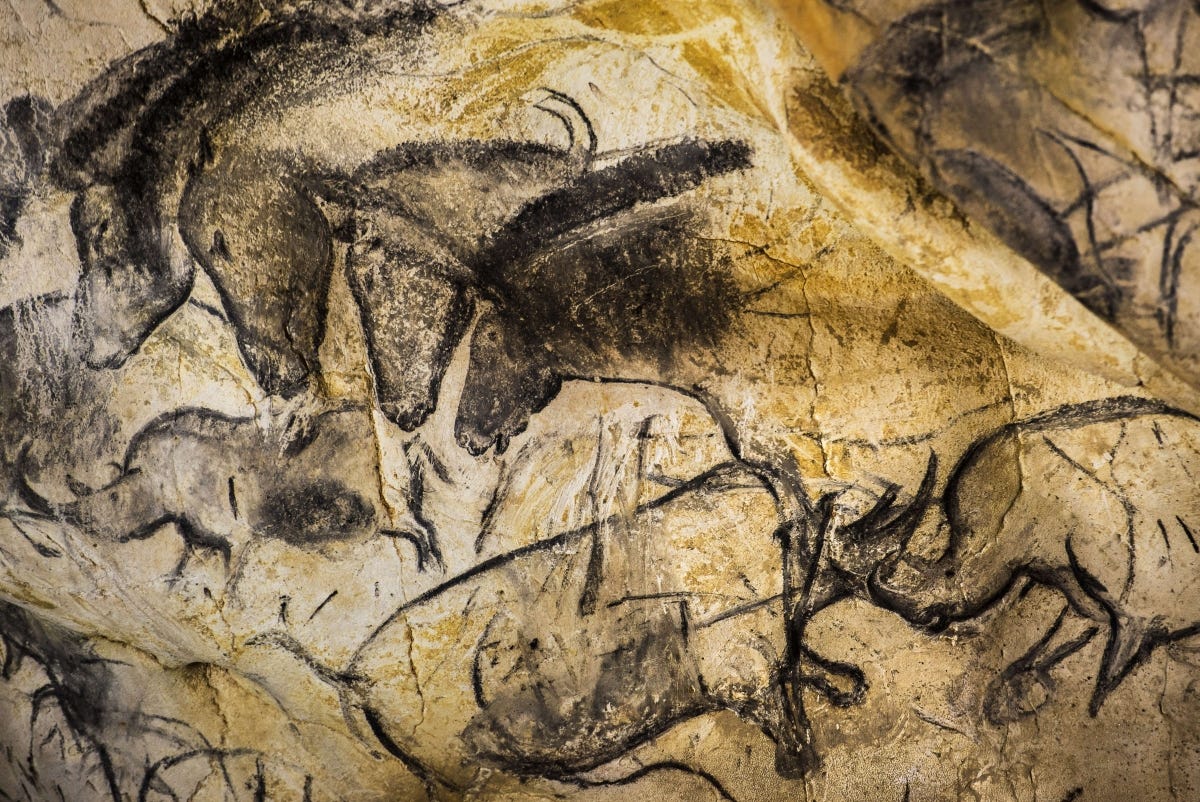The image depicts an abstract, horizontal cave painting or drawing etched onto a surprisingly smooth, wavy cave wall. The background of the cave wall is a blend of beige and yellowish hues. On the left side of the image, there are detailed sketches of four horse heads aligned in a vertical column, each shaded in dark brown or black, reminiscent of ancient carvings. The horse heads vary in size, with the first horse having a slightly more defined shape and a dark mane. Below the horse drawings, towards the lower portion of the image, there are two rhinoceroses facing and possibly fighting each other. Additionally, another rhinoceros appears off to the left of the horse heads, seemingly running. Overall, the other parts of the drawing appear somewhat blurry and less distinct but exhibit a cohesive theme of black and brown etchings against a yellowish cave wall backdrop.